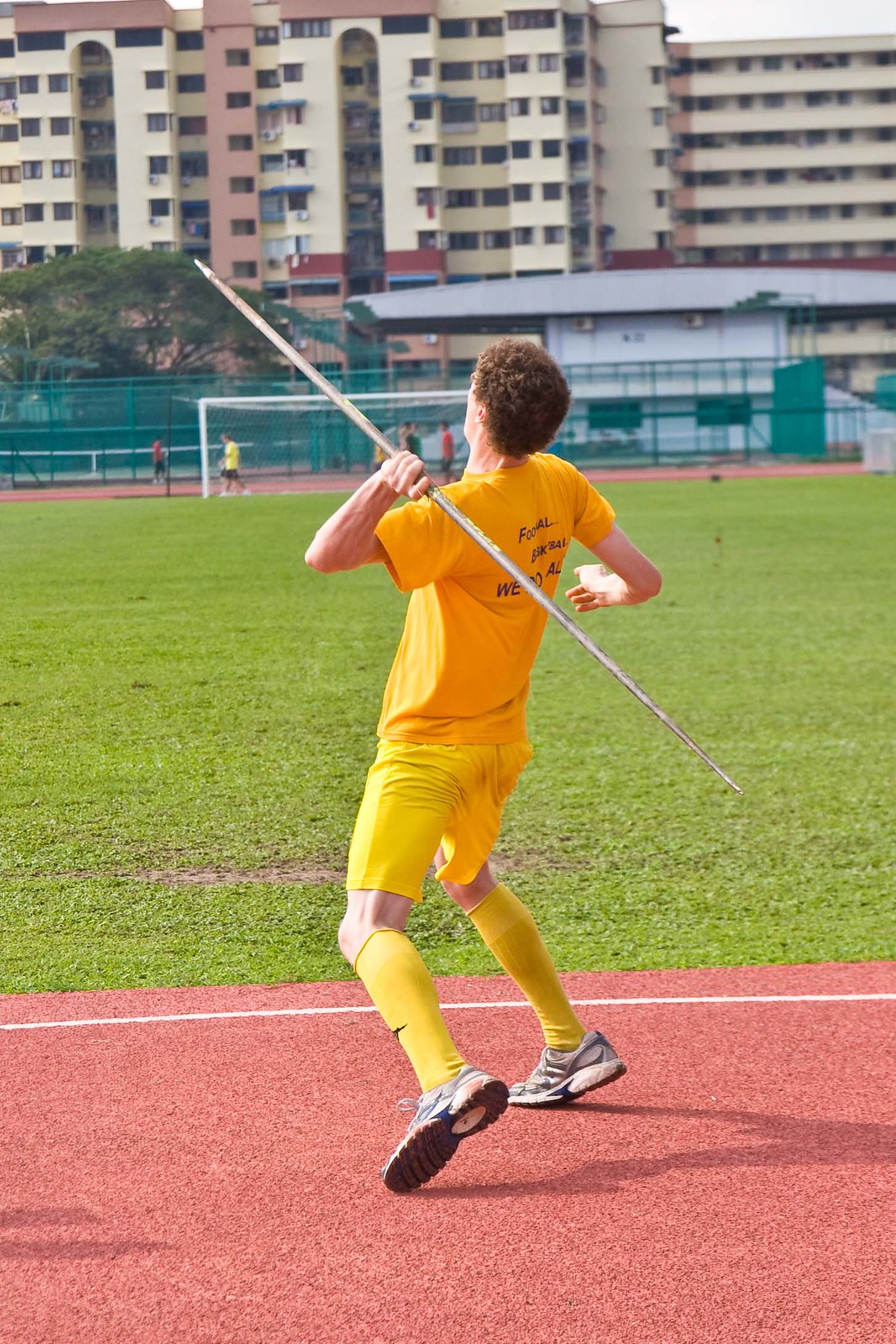This outdoor daytime photograph captures a young white man with curly hair, seen from behind, in the midst of preparing to throw a javelin on a track and field area. He stands on a green field, his left hand gripping the javelin as he readies to hurl it. The man is dressed in yellow: a slightly orange-tinged yellow t-shirt, yellow shorts, and yellow socks or shin guards. Though the complete text on the back of his shirt is obscured, partial letters suggest it reads something like "F-O-O...A-L...A, W-E, A-L."

In the background, to the left, a person in a yellow shirt and black shorts, and another in a red shirt and black shorts, can be seen walking near a soccer goal net. Further to the right, a group wearing red and black attire appears blurry due to their distance from the camera. Farther away still, a series of multi-storied buildings, likely residential or educational, rise against the skyline—predominantly gray with pink accents. Additionally, there are green fences and a set of spectator stands visible, enhancing the dynamic environment of the track and field area.